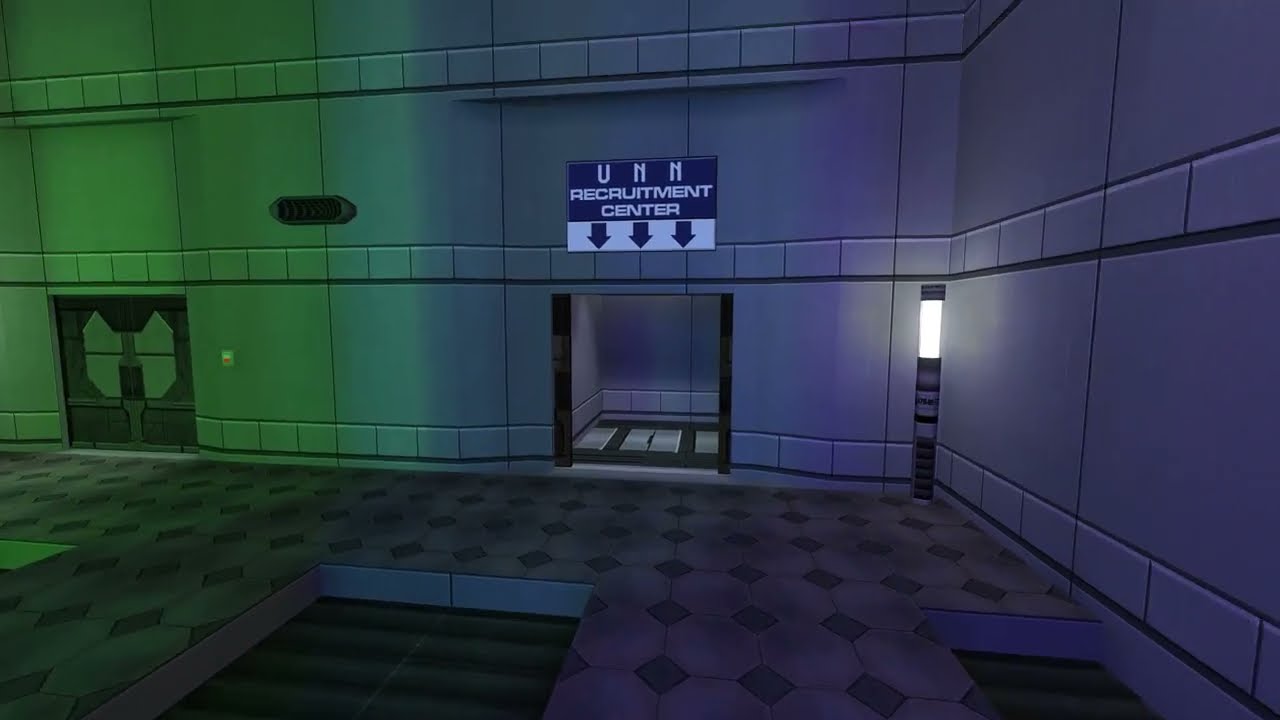The screenshot is from a video game, depicting the interior of a large, industrial, multi-story building with a distinct sci-fi aesthetic. The camera faces a wall made of large, wavy concrete panels that span multiple floors. The walls transition from a purplish-gray color on the right to a green hue on the left. Alongside this, the corridor corners are clearly demarcated with a light post in the right corner.

On the front wall is a prominently placed open doorway, above which a sign reads "UNN Recruitment Center" with three arrows pointing downwards to the door. The floor is tiled with repeating square patterns and smaller diamond shapes at the intersection points. There are also two rectangular depressions in the floor, which could be indicative of stairs or cages set into the ground, adding to the complexity of the room’s design. The futuristic setting is devoid of characters, focusing solely on the intricate details of the room's structure and lighting.